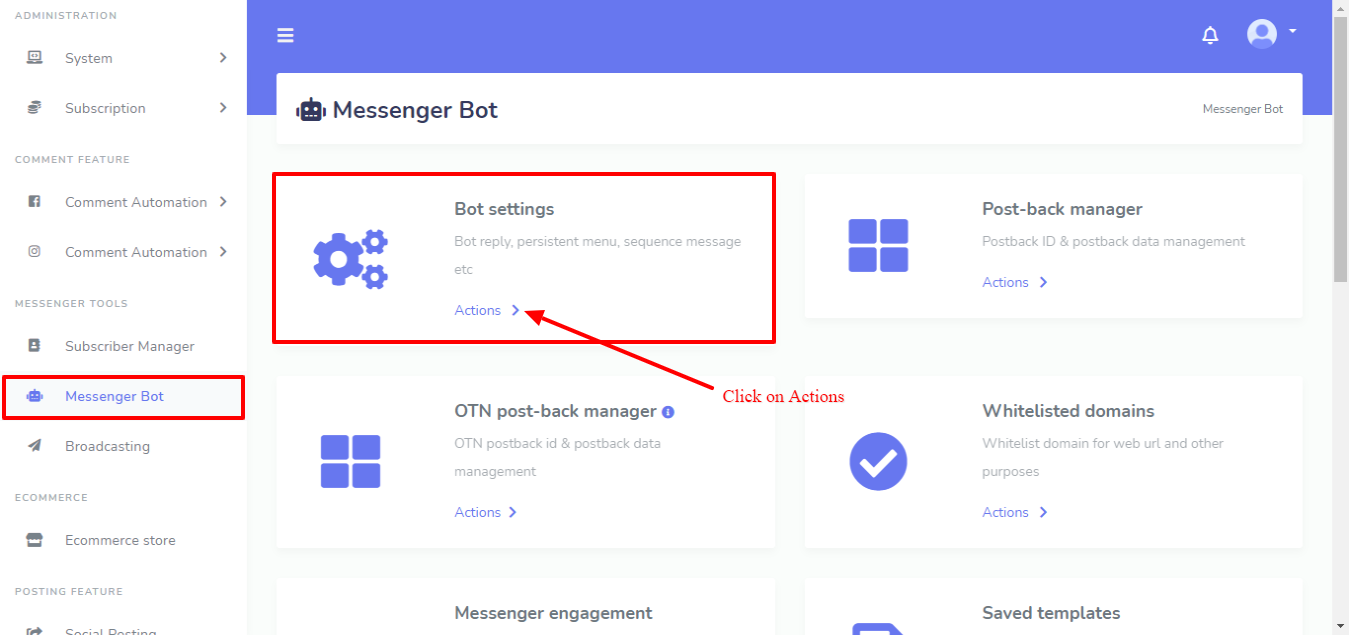The website features a prominent purple heading at the top. Below this, a white horizontal band spans the width of the page, displaying the text "Messenger Bot" alongside an image of a robot's head. A red-outlined box labeled "Bot Settings" is highlighted with a red arrow pointing towards it. Directly beneath this, the text "OTN Post-Back Manager" is displayed, with a note to "Click on Actions" at the end of the arrow.

At the top of the page, "Post-Back Manager" is clearly labeled, followed by "Actions" which can be clicked. Below, "Whitelisted Domains" is mentioned with a description reading "Whitelist domains for web and other purposes," with the actions option in purple, which is also clickable. Further down, partially obscured text mentions "Messenger Engagement" and "Save Templates," with the latter being cut off.

On the left-hand side of the screen, a vertical menu lists several options: "System Subscription," "Comment Automation" (repeated), "Subscriber Manager," "Manage Bot" (in a red-outlined box), "Broadcasting," "E-Commerce Store," and another cut-off item at the bottom.